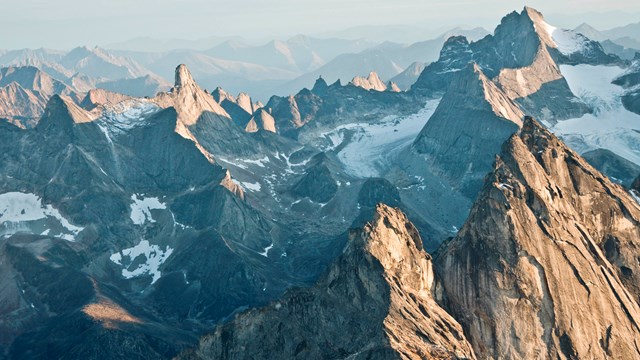The photograph captures a sprawling, mountainous landscape, likely taken from an airplane. Dominating the frame are stony, sharp-peaked mountains, primarily gray with patches of brown, interspersed with white snow. In the foreground, particularly on the right side, two prominent, sharp peaks stand out, devoid of snow. Just behind these peaks, there is what appears to be a glacier, with heavy snow nestled in the adjacent valley. The left side features slightly lower peaks with scattered snow. This vista extends all the way to the horizon, where the mountains gradually taper off. The sky above is a uniform gray, suggesting a haze possibly from fog or pollution, despite the daytime light casting visible shadows. The entire scene is devoid of any human presence or greenery, reinforcing a sense of remote, untouched wilderness, perhaps in the summer months given the sparse snow coverage on some of the peaks.